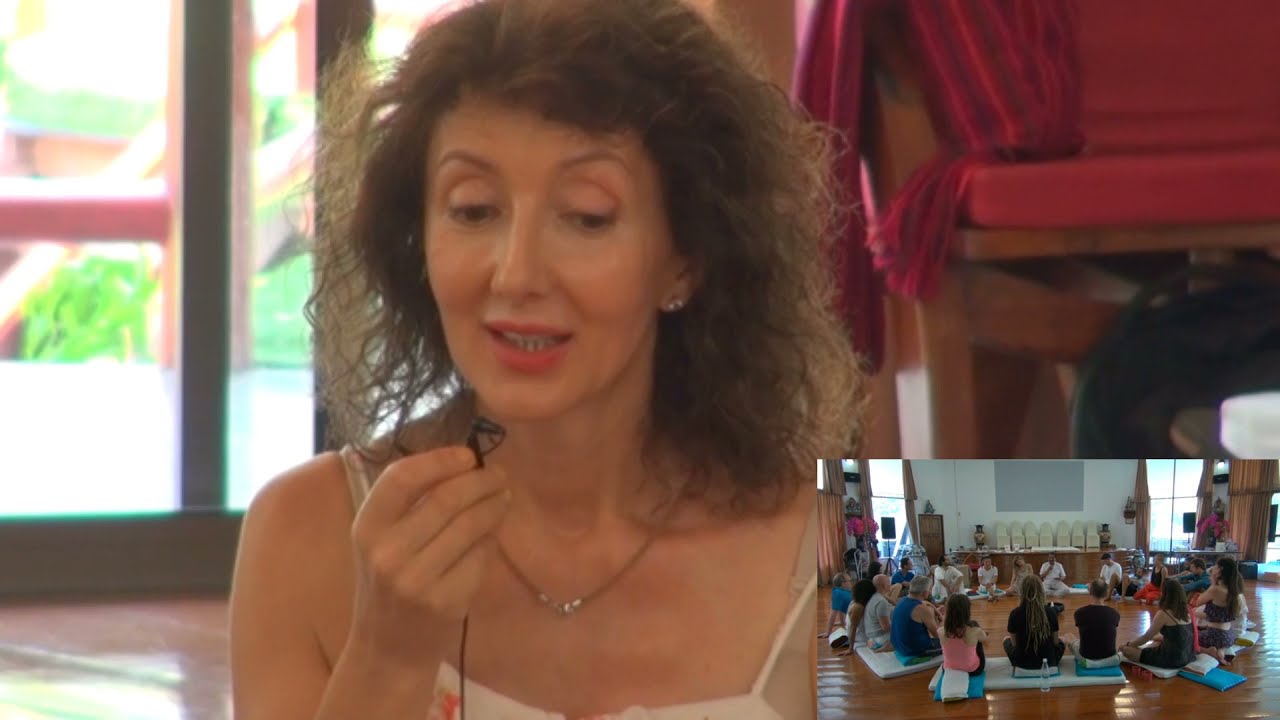The image is a detailed, color landscape photograph depicting a woman with medium-length, messy, dark brown hair, wearing a white tank top and a gold necklace. She is positioned slightly to the left of the center and appears to be speaking into a small, wired microphone held close to her mouth. Behind her, there is a door with black window panes and some furniture, including a table or cabinet draped with a red curtain on the right side. In the lower right corner of the photograph, there is a smaller inset image showing a group of people sitting in a circular formation on a shiny brown floor, which seems to be a classroom or a retreat environment. The people are on mats or pillows and dressed in casual or gym attire. The scene suggests that the woman is possibly teaching or leading a session, potentially communicating with the group via a video feed or conference setup. The overall style of the photograph is freeze-frame video or photo realism.